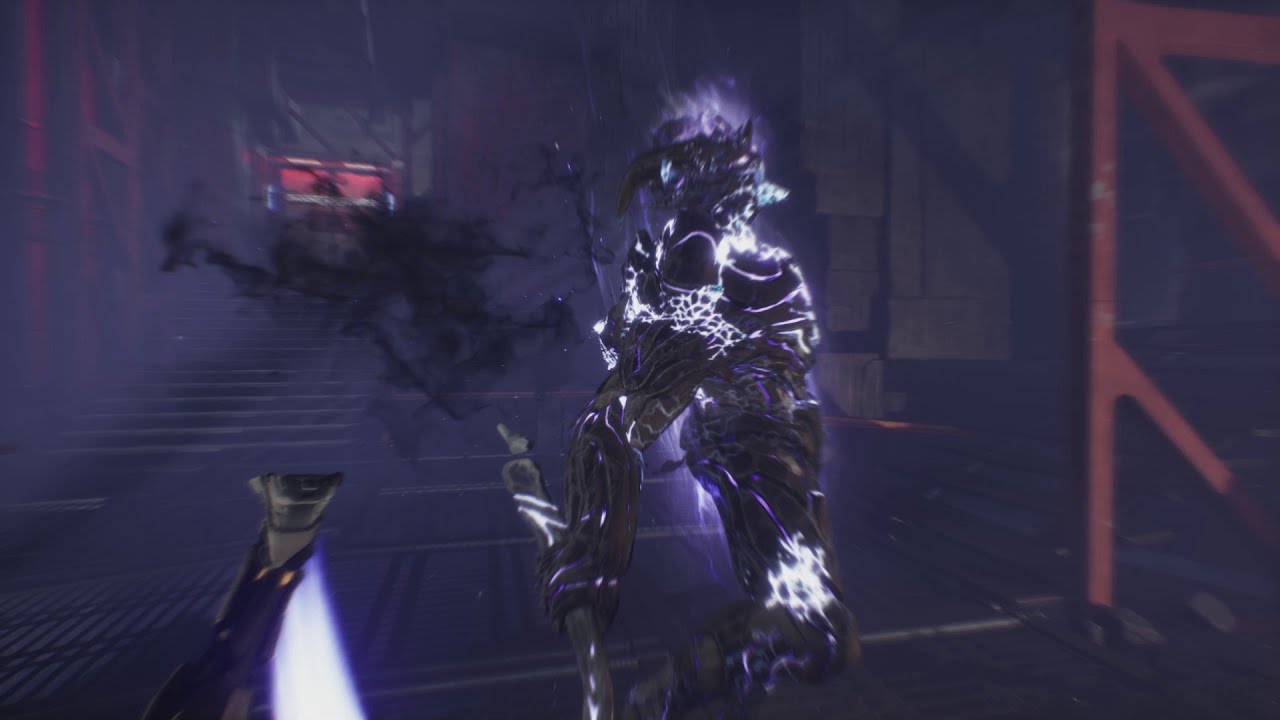In this somewhat blurry, horizontally aligned rectangular image from a video game, a central creature commands attention. This figure, potentially a monster or alien, features dark, thick muscles with intricate blue and white glowing striations. Its overall coloration blends browns and blacks with hints of metallic purple, giving it a textured, armored appearance. Facing towards the right, it holds a spear-like weapon in its right arm, while something partially obscured occupies its left arm. 

Strikingly, the creature appears to be in the midst of an electrical attack, with light permeating various parts of its body, enhancing its menacing presence. The backdrop, though blurred, suggests an industrial setting, possibly a warehouse, with red railings and wooden elements. A splatter of black behind the creature adds to the chaotic scene. Additionally, a faint image of another possible creature or weapon with a beam of light emerges from the far left, hinting at a potential conflict. The overall scene is tinged with dark grays and purples, intensifying the ominous atmosphere.